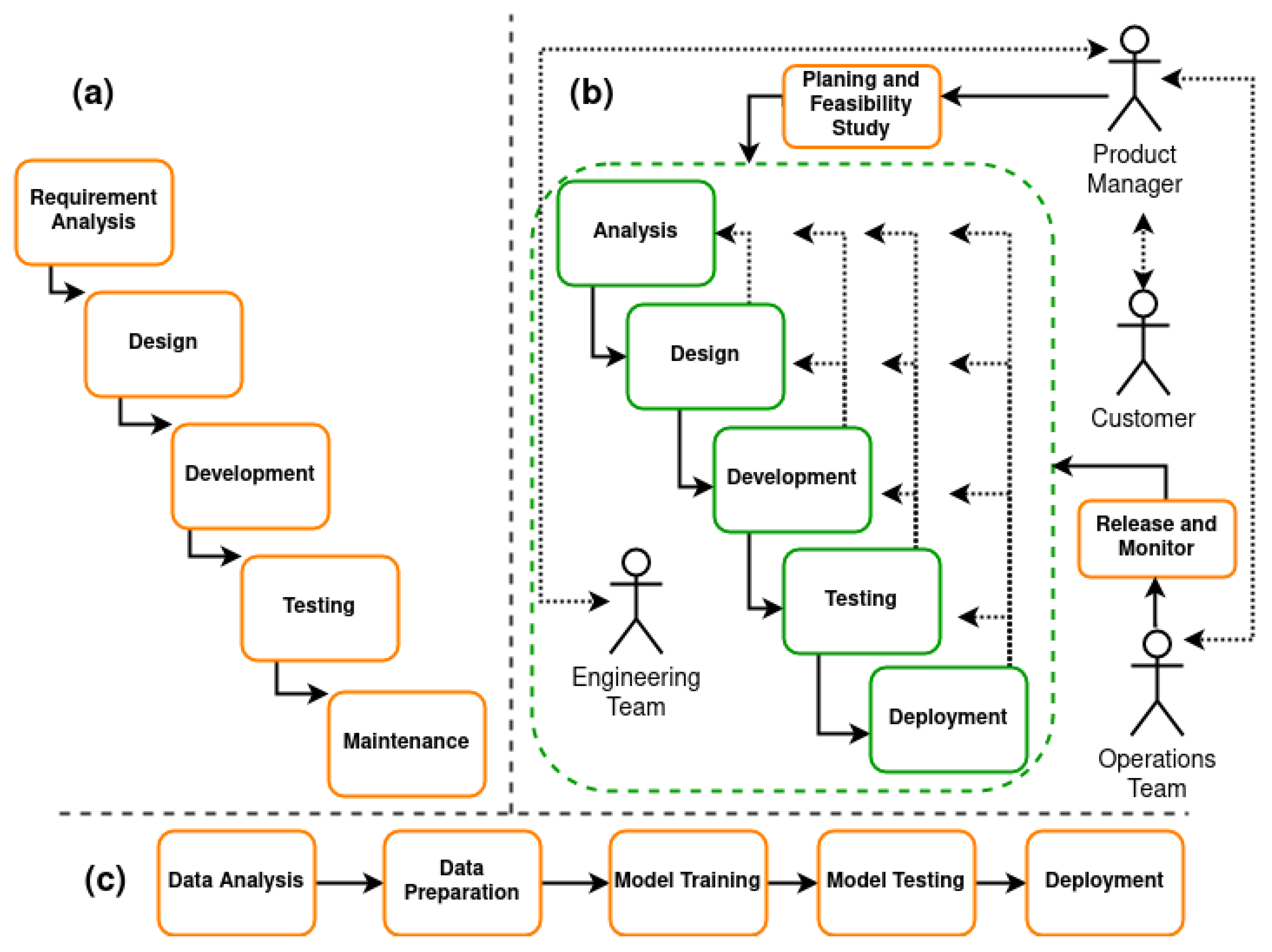The image presents a comprehensive, color-coded flowchart divided into three distinct sections labeled A, B, and C. 

Section A, located on the left, outlines a sequential process in a series of step-like orange-colored boxes with white text. It begins with "Requirement Analysis" at the top, progressing through "Design," "Development," "Testing," and concluding with "Maintenance" at the bottom. 

Section B, positioned on the right, highlights the interactions and roles of various stakeholders, including the "Product Manager" at the top right, "Customer," "Operations Team," and "Engineering Team." The green boxes depict stages such as "Planning and Feasibility Study," "Analysis," "Design," "Development," "Testing," and "Deployment," with arrows illustrating the flow and connections between these roles and steps. Additionally, various stick figures represent the stakeholders involved, with arrows pointing leftward and rightward to show their interactions.

Section C, located at the bottom, details the data-related workflow in orange boxes, starting with "Data Analysis" on the left, followed by "Data Preparation," "Model Training," "Model Testing," and culminating in "Deployment" on the right. 

Overall, the flowchart meticulously maps out the processes, roles, and interactions involved in both the development and data analysis workflows, with distinct colors and labeled sections for clarity.